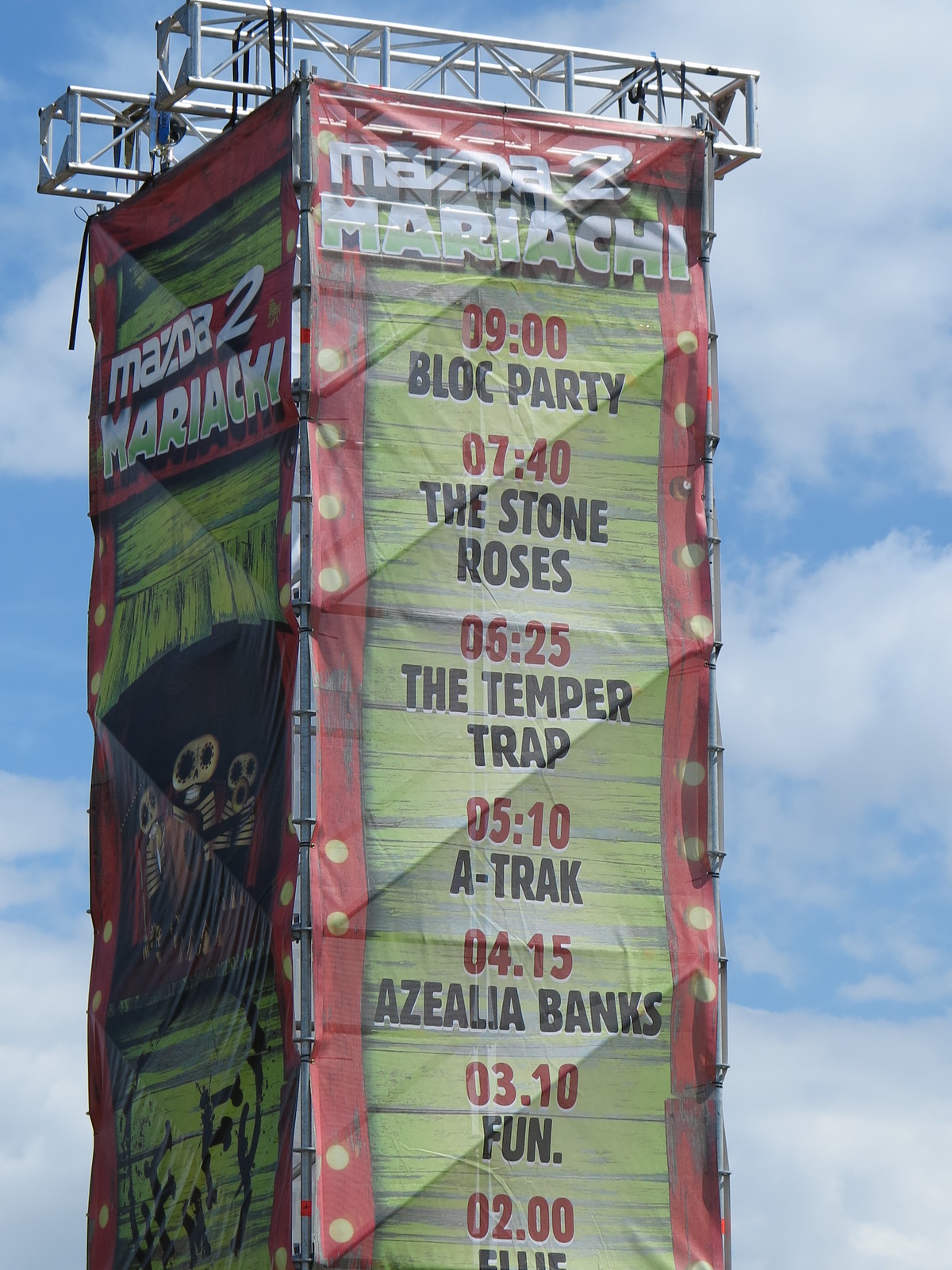The photograph features an impressively tall metal tower, wrapped entirely in large, colorful banners. The structure, reminiscent of scaffolding with pipes that frame buildings under renovation, towers into a clear blue sky dotted with white clouds, indicating it's daytime. Dominating the banners are bold, vibrant hues of red, yellow, green, and white, with meticulously detailed event information.

At the pinnacle of the banner, the text "Mazda 2 Mariachi" prominently stands out, suggesting a recurring theme or headliner. Below this heading lies a vertical array of event schedules, marked by black fonts for artist names and red fonts for times. The schedule reads: 0900 Block Party, 0740 The Stone Roses, 0625 The Temper Trap, 0510 A-Track, 0415 Azalea Banks, 0310 Fun, and 0200 Ellie (partially visible).

The left portion of the banner mirrors the main heading, "Mazda 2 Mariachi," and features an animated stage design with green-colored curtains, evoking a music festival atmosphere. The tower’s signage and its elaborate decor strongly indicate it's a key feature of a vibrant, multi-artist event, celebrating various musical acts throughout the day.